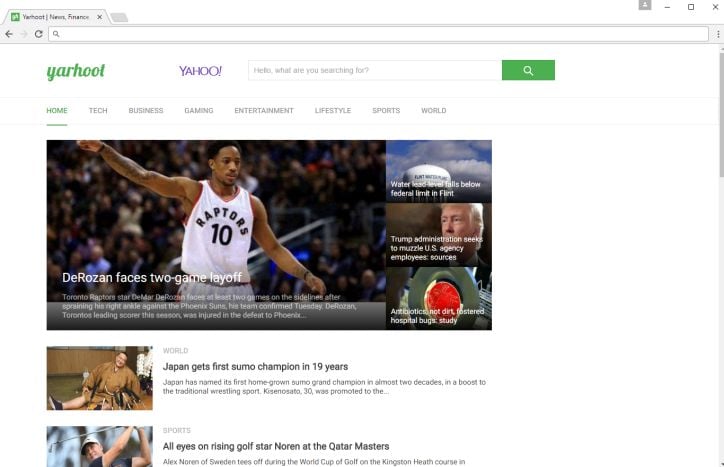This detailed caption describes a web page layout for a fictional news website named "Yaarhoot," closely resembling Yahoo News. The webpage header prominently displays the "Yaarhoot" logo in green font on the left, adjacent to the classic purple "Yahoo" logo. At the center of the header is a search bar with placeholder text that reads, "Hello, what are you searching for?" and a green search button to the right.

Beneath the header is the navigation bar that lists the main categories: Home, Tech, Business, Gaming, Entertainment, Lifestyle, Sports, and World. This organized setup allows users to effortlessly browse through different sections of the site.

The main content area is artistically divided, with a large featured article on the left and three smaller articles stacked vertically on the right. The featured article spotlights a basketball player, DeMar DeRozan of the Toronto Raptors, wearing jersey number 10. The headline "DeRozan Faces Two-Game Layoff" is prominent, with subtext elaborating on his suspension due to a conflict with a referee.

The smaller articles include a range of topics: 
1. An image of a water tower accompanies a headline about water contamination.
2. A close-up of a man in a suit paired with the headline, "Trump Administration Seeks to Muzzle U.S. Agency Employee Sources."
3. An image of Petri dishes with the headline, "Antibiotics Often Not Needed for Hospitalized Kids: Study."

Additional sections highlight world news and sports news, all within a clean and organized layout that ensures ease of navigation and readability for users.